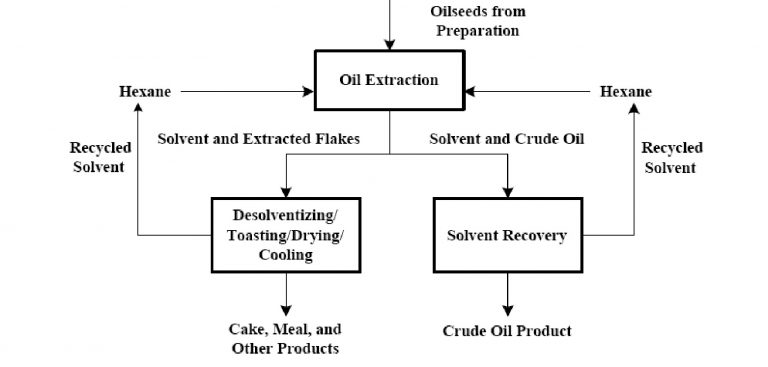This detailed, black and white flowchart visually represents the process of oil extraction. At the top, an arrow from the text "oil seeds from preparation" leads down to a large, highlighted black rectangle labeled "oil extraction." This central rectangle has multiple inputs and outputs. Arrows labeled "hexane" point into it from both sides, fed by "recycled solvent" arrows looping back from other parts of the chart. 

From "oil extraction," the chart splits into two main pathways. On the left, an arrow leads to a black rectangle that reads "desolventizing, toasting, drying, and cooling," which then points downward to "cake, meal, and other products." On the right, the flow moves through "solvent and crude oil" into a rectangle labeled "solvent recovery," which subsequently transitions to "crude oil product." 

Additionally, the right pathway has a feedback loop where "solvent recovery" arrows cycle back up to the main "oil extraction" process, completing the feedback loop of "recycled solvent" transforming back into "hexane."

This graph is digitally created, featuring a simple yet precise layout with clearly defined connections and relationships between each stage of the oil extraction process. The clean, minimalistic design ensures focus on the informational flow, with a majority of the visual space dominated by a solid white background contrasted by black text and lines.